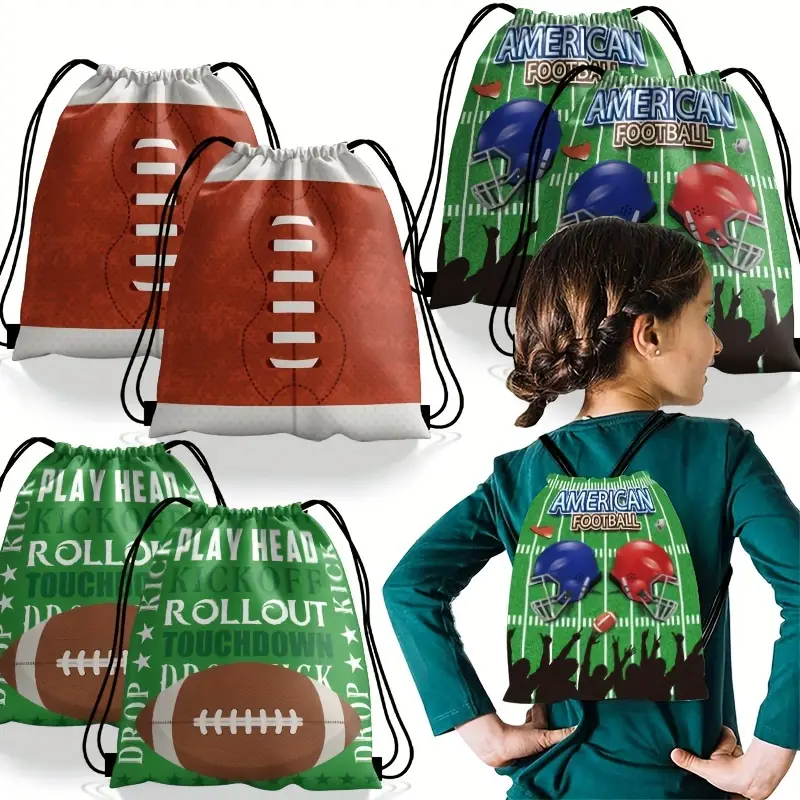This advertisement features a young girl, approximately 10 or 11 years old, standing in the lower right corner with short brown hair. The girl, who appears cute and caucasian, is wearing a teal long-sleeve shirt and a dark green jersey. Her hair is styled in a braid behind her head. She is showcasing a drawstring backpack designed with a green football field background that prominently displays "American Football" in blue and beige text, accompanied by illustrations of blue and red helmets and a football. 

The image also highlights other backpack designs: one adjacent to the girl features a lighter green color adorned with football-related words like "play," "head," "kickoff," "rollout," and "touchdown" in various colors, and a football illustration at the bottom. Another design visible in the top left of the frame resembles a brown pigskin football complete with white laces at the center, emulating the look and texture of an actual football. The overall theme of the backpacks revolves around American football, targeting children as the primary audience for these sporty, decorative carry bags.